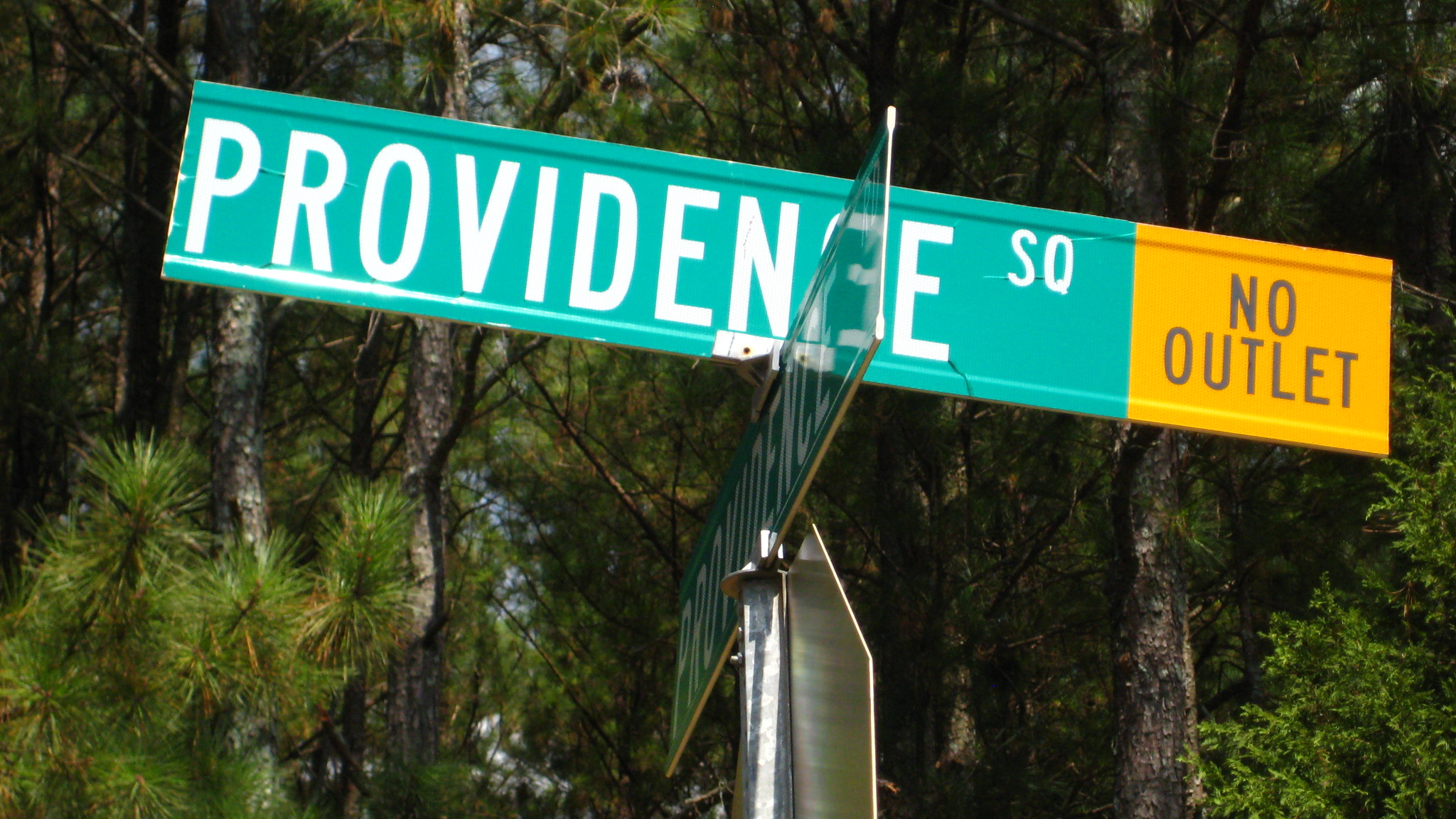The color photograph, taken in landscape orientation, captures a close-up of a street sign at an intersection in an outdoor setting, likely a residential area. The prominent street sign in the center features an aqua background with white letters spelling out "Providence SQ," denoting Providence Square, and a dark gold portion to the right with gray letters proclaiming "NO OUTLET." Below this sign, another sign appears, although partially obscured and slightly sideways, hinting at a stop sign due to its octagonal shape. The entire sign assembly is mounted on a silver pole. In the background, a dense cluster of trees dominates the scene, including both pine trees and various other kinds, with tree trunks forming a natural backdrop. A glimpse of something white—a possible house or building—can be seen faintly through the trees.